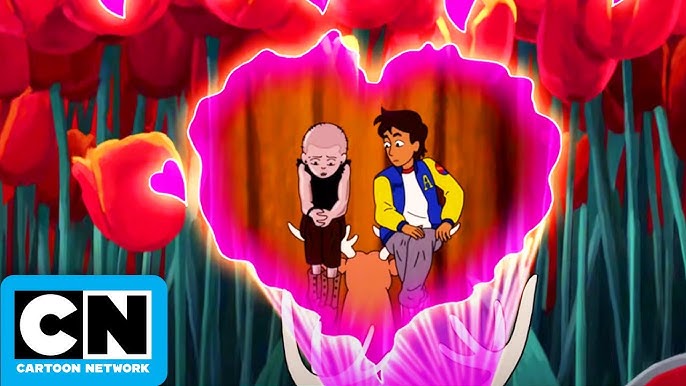This animated still from Cartoon Network features a colorful background dominated by large tulips with visible stems. Most of the tulip tops are positioned near the top of the frame, except for a few lower ones on the left, including one with a purple heart. Central to the image is a heart-shaped, open tulip containing two figures. On the left is a young boy with a distressed expression, short hair, wearing black clothes, with his hands clasped together. To his right is a slightly older boy with brown skin, dark hair, wearing gray pants, a white T-shirt, and a blue and yellow jacket. His eyes are open, looking with concern at the younger boy. The scene is set against a backdrop of strange, vibrant flowers. In the lower left corner of the frame is the Cartoon Network logo, featuring a large "C" and "N" in alternating black and white boxes, with "Cartoon Network" written beneath it.